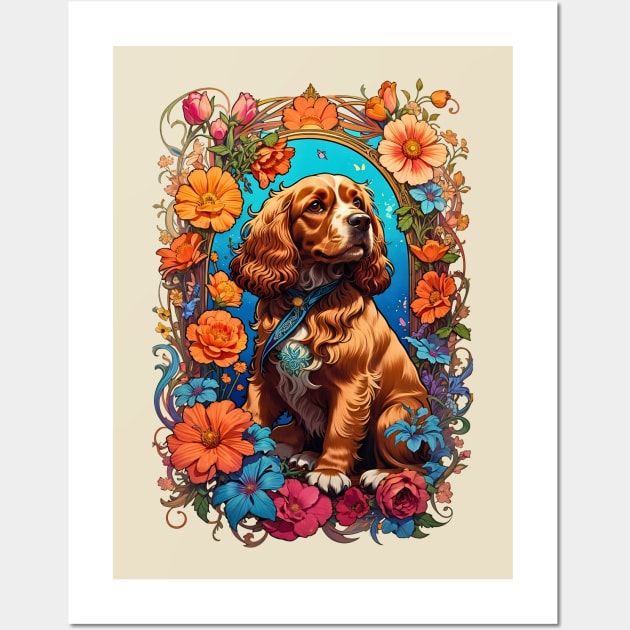The image features a richly detailed portrait of a dignified brown cocker spaniel, accentuated with various distinctive markings such as a white chest, white toes, and a white stripe running from the top of its head down to its mouth. The dog appears to be gazing slightly upwards and to the right as if looking at its master, creating a tender and affectionate atmosphere. Encircling the dog is an ornate, woven oval wreath of vibrant flowers—including roses, tulips, and daisies—in hues of blue, red, fuchsia, orange, and pink, interspersed with vines and leaves. This floral frame is set against a calming turquoise-blue background adorned with delicate butterflies. The entire artwork is presented within a white rectangular frame with a light gray mat, suggesting the owner or artist's fondness for this beloved pet.